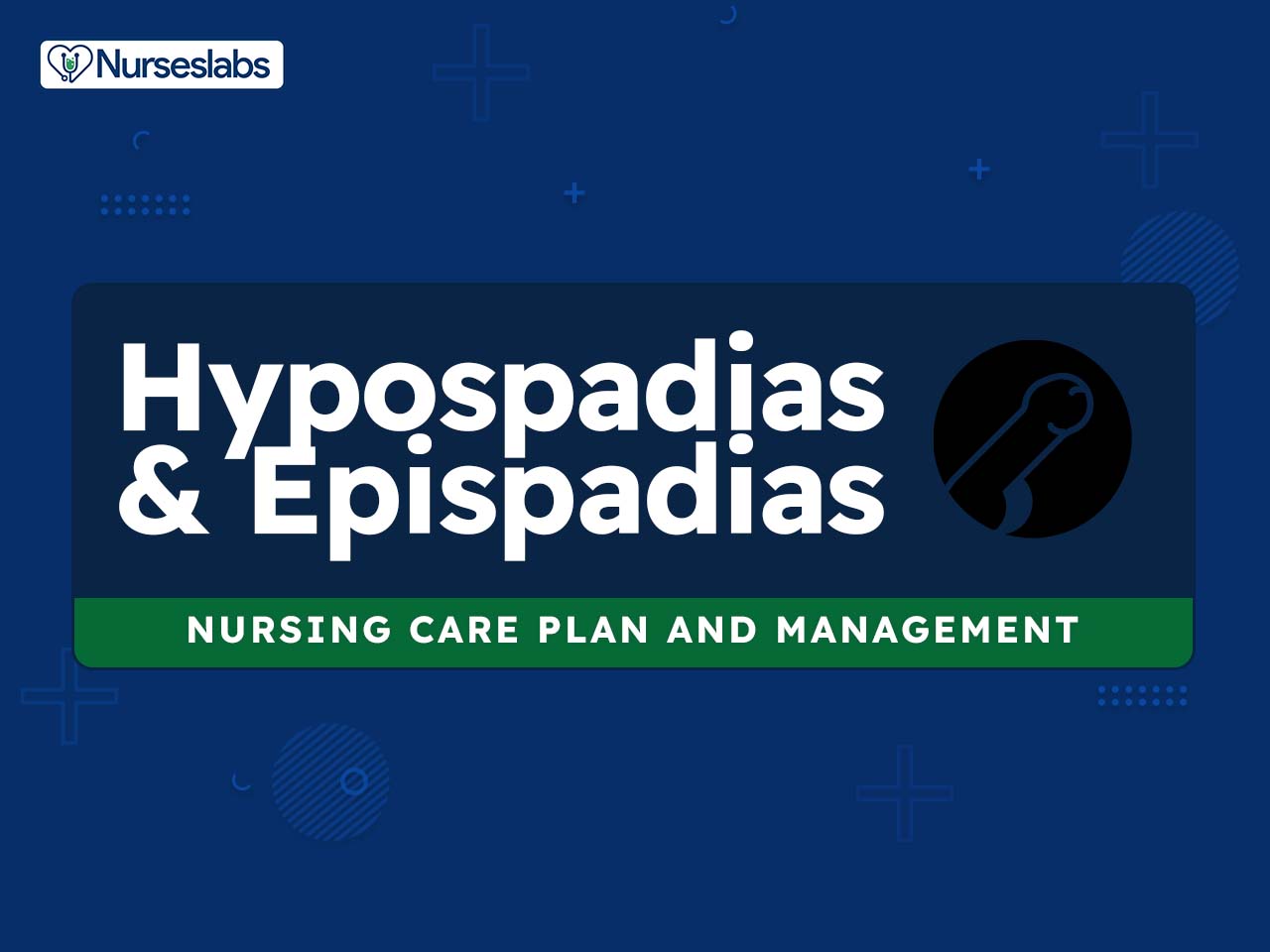The image appears to be an informational sheet or advertisement, possibly the first page of a presentation or document. It features a blue square background adorned with various medical symbols, including crosses, dots, and crescents. In the top left corner, "Nurses Labs" is prominently displayed in white text, accompanied by a heart icon formed by a stethoscope. The center of the image showcases a darker blue text box with the white text "Hypospadias and Epispadias," indicating the medical conditions being addressed. To the right of this text, there's an illustrative drawing of a penis, emphasizing the urological focus of the content. Below, a green strip features the text "Nursing Care Plan and Management" in white, signifying the purpose and target audience of the document.